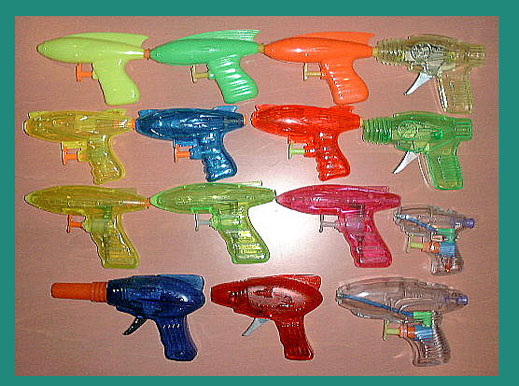This is a detailed photograph of 16 colorful toy squirt guns, all mounted in a grid on a dusty pink wall. The squirt guns, each designed in a revolver style, showcase a wide spectrum of colors. The top left gun is lime green, below it is a transparent yellow, followed by a transparent green, and finally a blue gun with a red tip. To the right, the sequence on the top row includes a green gun, a blue one, a transparent green, and a semi-transparent red gun. The sequence is repeated, showing an orange gun, a red gun, a transparent pink, another transparent green gun, a brighter green, and two clear guns. The intricate background features a green border and a brown rectangle within, accented by a gradient of white to tan and finally to brown, centered by a white spot. The squirt guns are subtly iridescent, displaying hues of blue, purple, red, and lavender, and are all pointed in the same direction.